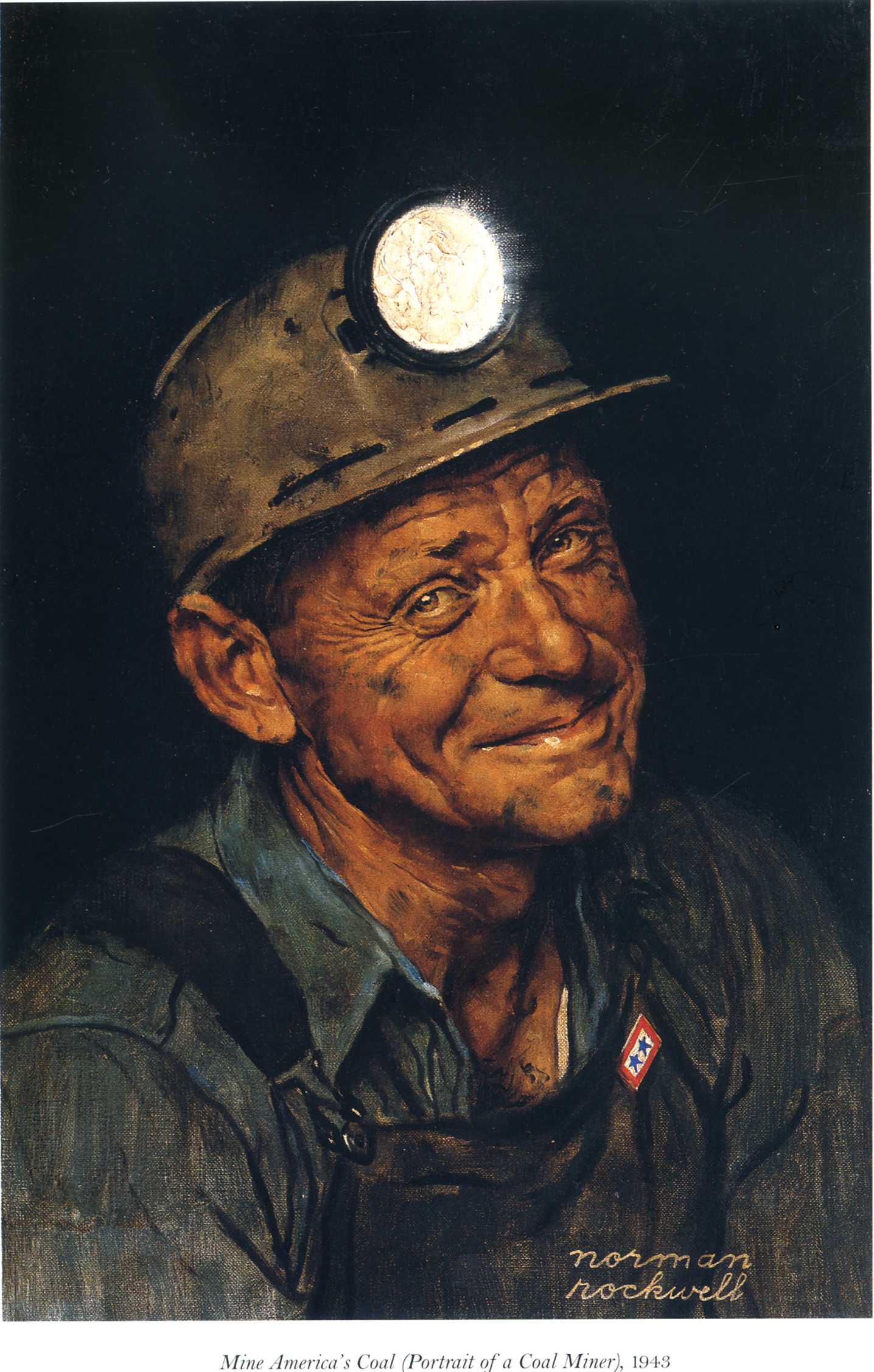This detailed Norman Rockwell painting, "Mine America's Coal: Portrait of a Coal Miner, 1943," vividly showcases a middle-aged Caucasian coal miner covered in black soot. The miner is depicted with a well-worn, helmet-like hat adorned with a headlamp that's turned on. His attire includes overalls with visible straps and a blue shirt, heavily darkened by coal dust, over a barely visible dirty white t-shirt. His miner number, 55, appears on his overalls. The man’s face is marked by deep wrinkles, crow’s feet around his eyes, and a large, uneven nose, all conveying a lifetime of hard work in the mines. His eyes, either brown or blue, twinkle kindly as he smiles with his mouth closed, revealing a gentle demeanor. His thin, short hair, prominent Adam's apple, and a slightly misshapen right ear further contribute to the realism of his character. The portrait, set against a completely black background, emphasizes the miner's presence. Rockwell's signature is visible in the lower right corner, solidifying the authenticity of this powerful depiction of America's working class.